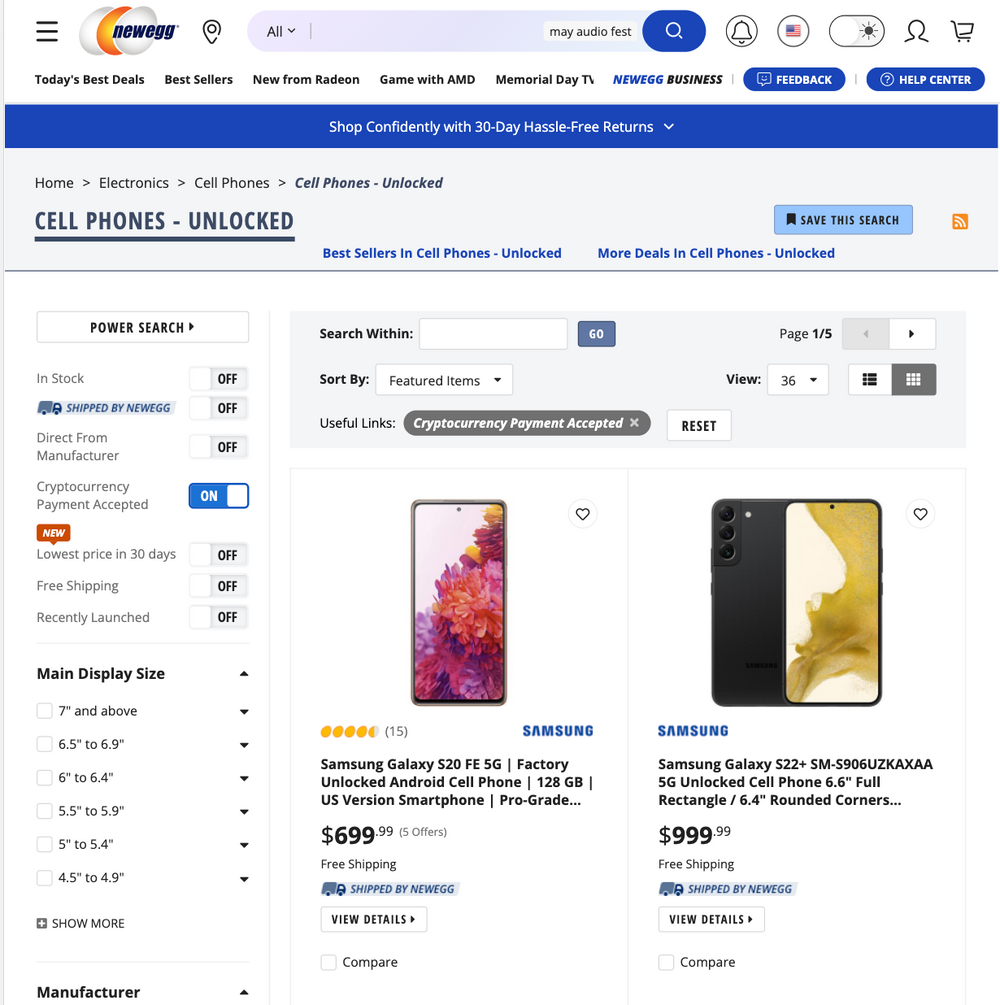The screenshot captures the Newegg website, focusing on its top navigation and featured products. In the upper left-hand corner, the recognizable Newegg logo is prominently displayed. Directly to the right, there is a search bar for easy access to product searches. Adjacent to the search bar are several icons, including a notifications menu, a language selection option set to English, and a toggle button for switching between dark and light screen modes.

Below this primary navigation area is a horizontal menu listing various sections such as "Today's Best Deals," "Best Sellers," "New from Radeon," "Game with AMD," and a seasonal "Memorial Day" section. Additional links for "Newegg Business," "Feedback," and the "Help Center" are also present.

The screenshot features two highlighted products below the navigation bar. The first product is a Samsung Galaxy S20 FE 5G, described as a factory-unlocked Android cell phone with 120GB of storage, priced at $69.99. To the right, another product is listed—the Samsung Galaxy S20 II, an unlocked cell phone priced at $99.99.